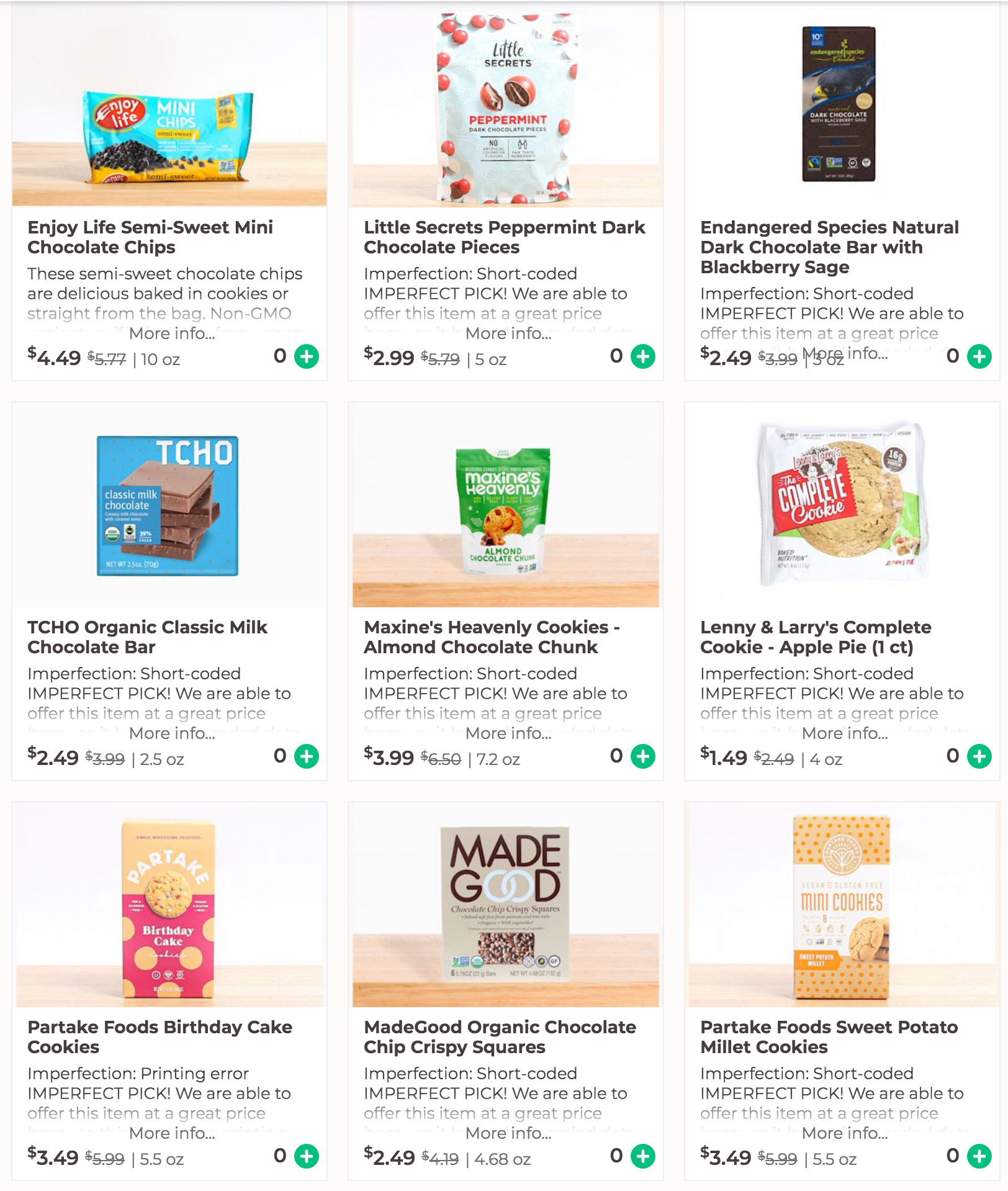**Detailed Image Caption:**

The screenshot displays a list of 9 products organized in a 3 by 3 grid on a website. Each product entry follows a consistent format: a rectangular image appears at the top, followed by a bolded title, a truncated description, and other key details.

1. **Enjoy Life Semi-Sweet Mini Chocolate Chips**
   - **Description**: These semi-sweet chocolate chips are delicious baked in cookies or straight from the bag, non-GMO. The rest of the description is cut off.
   - **Pricing**: Original price $5.77, discounted to $4.49.
   - **Size**: 10 oz.
   - **Quantity Control**: Bottom right features a bolded zero with a green circle containing a white plus sign for adding items.

2. **Little Secrets Peppermint Dark Chocolate Pieces**
   - **Description**: Imperfection Short Coated Imperfect Pink. We are able to offer this item at a great price.
   - **Pricing**: Original price $5.79, discounted to $2.99.
   - **Size**: 5 oz.
   - **Quantity Control**: Similar to previous.

3. **Endangered Species Natural Dark Chocolate Bar with Blackberry Sage**
   - **Description**: Imperfection Short Coated Imperfect Pick. We are able to offer this item at a great price.
   - **Pricing**: Original price $3.99, discounted to $2.49.
   - **Size**: 3 oz.
   - **Quantity Control**: Similar to previous.

4. **TCHO Organic Classic Milk Chocolate Bar**
   - **Description**: The description is not visible in the screenshot.
   - **Pricing**: Pricing details are not visible.
   - **Size**: Size detail is not visible.
   - **Quantity Control**: Similar to previous.

  The same pattern continues for the remaining five products: a rectangular image at the top, followed by a bolded title, a truncated description, original price crossed out with the current price, size, and a quantity control feature. The website design follows a uniform layout with a white background, bolded titles, greyed-out truncated descriptions, and a distinctive green plus sign within a circle for adding products to the cart.